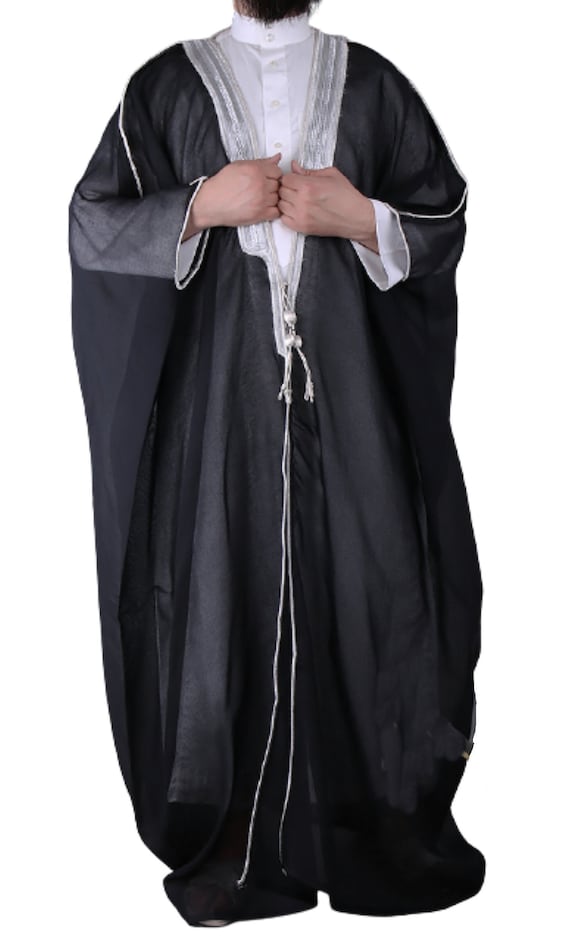The image depicts a man dressed in what appears to be a priestly or pastor's robe, standing against an entirely white background. The figure's face is not visible, but a beard at the lower chin level can be seen. The man is adorned in a long black robe that reaches down to cover his feet, leaving them out of sight. A distinctive white buttoned collar encircles his neck, complemented by white buttons extending down towards the waistline. The robe features a V-shaped section at the chest, outlined with a silver-white trim adorned with hanging beads. Running vertically along the robe, there is a thin silver stripe that adds to the garment's intricate detailing. White lining is visible around the collar and cuffs, as well as a thin white stripe along the arms. The person's arms are raised, with hands positioned near the chest, making it possible to see a few veins on his hands.